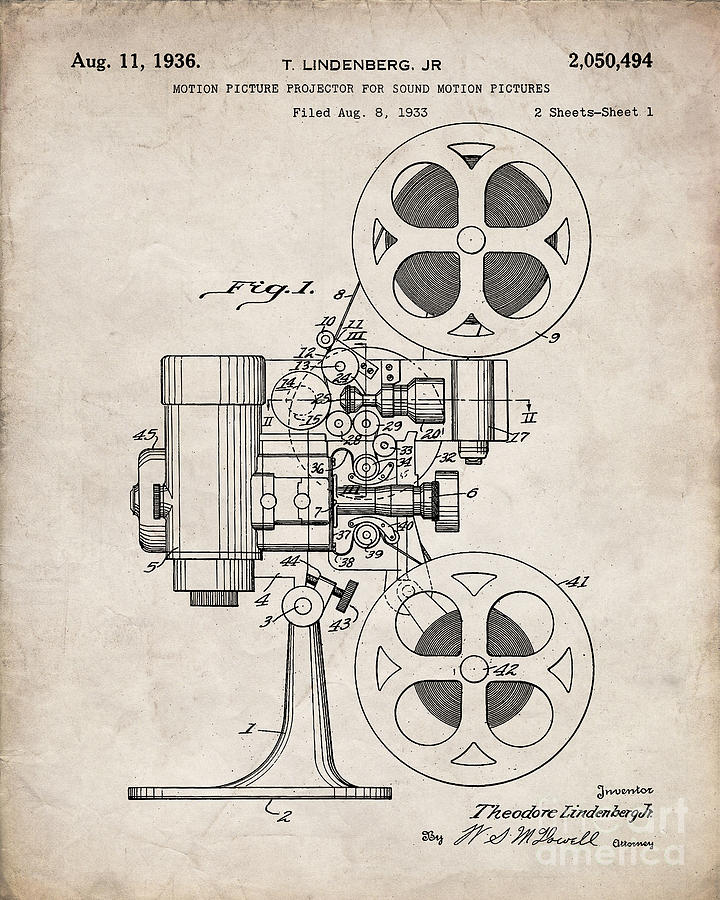The image depicts a detailed schematic of an old motion picture projector, likely a sound motion picture projector. Drawn on yellowed, weathered paper, the schematic features intricate illustrations of the machine, including two film reels—one at the top and one at the bottom—with a complex mechanism in between. Arrows and numbers label various components of the device. The text on the image states, "August 11, 1936," with a patent number "2,050,494" in the top right. It identifies the inventor as "T. Lindenburg, Jr." and notes the filing date as "August 8, 1933." The bottom right corner bears the name "Theodore Lindenburg" with a cursive signature of the attorney, "W.S.M. Dowell." The schematic is centered in the image, emphasizing the central mechanism of the projector. This appears to be an original patent drawing, capturing both the technical intricacies and historical context of the invention.